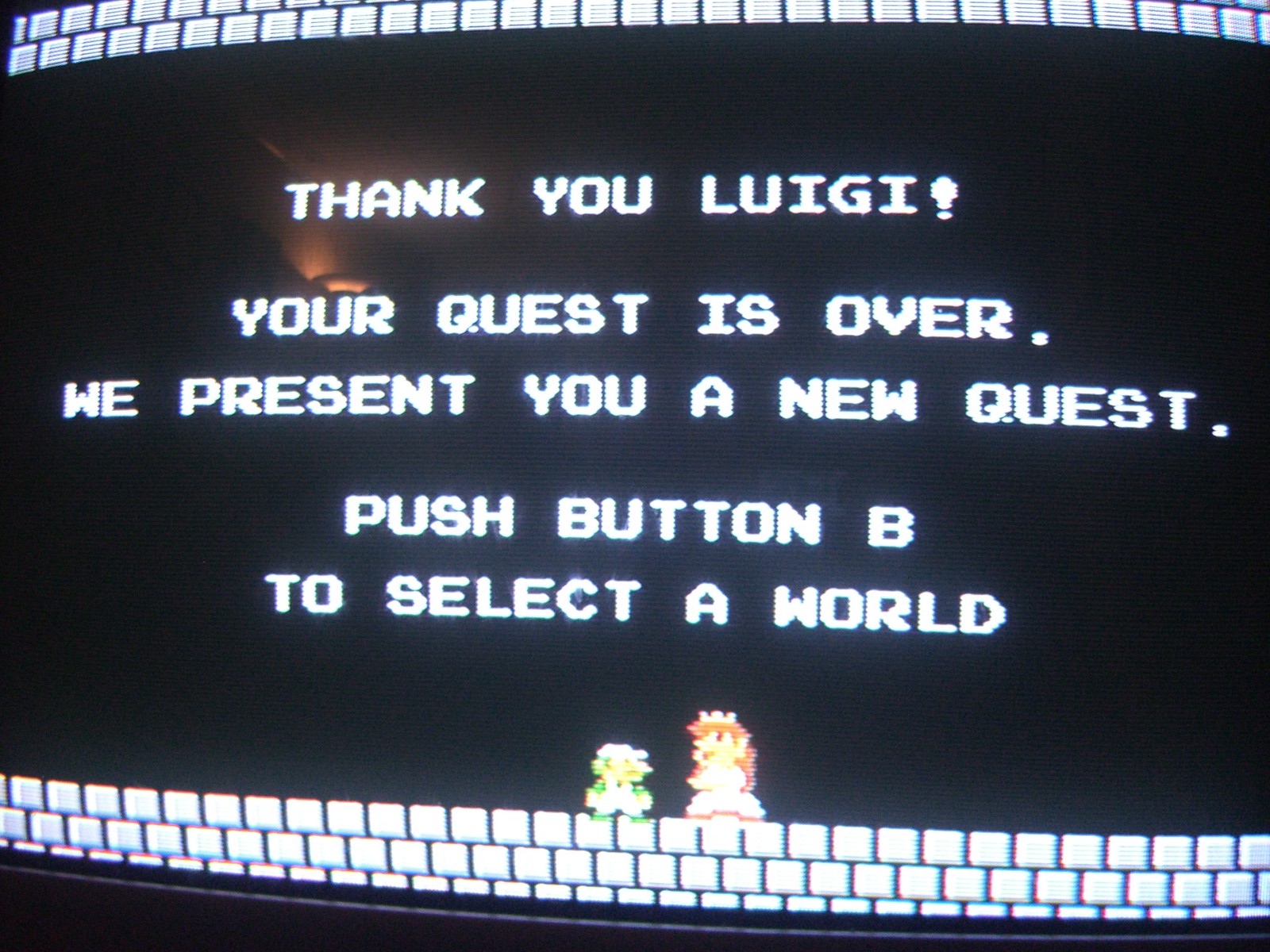The image is a photograph of an old computer monitor displaying a scene from the original Super Mario Bros. game on the Nintendo Entertainment System. The screen, which has a slight curvature indicative of vintage monitors, shows the end of a level with black background and both the top and bottom bordered by rows of white bricks. The text on the screen reads: "Thank you, Luigi! Your quest is over. We present you a new quest. Push button B to select a world." Prominently displayed at the bottom-center of the screen are two classic characters, Luigi and Princess Peach, who are slightly blurred. Luigi, dressed in a white cap, green shirt, and white overalls, stands shorter than Princess Peach, who is adorned in a pink dress with a flowing brown hair and a crown. They are positioned in what appears to be a castle setting, adding a nostalgic touch to this iconic video game moment. A reflection of a lamp can be seen in the upper left corner, further emphasizing the photo's vintage aesthetic.